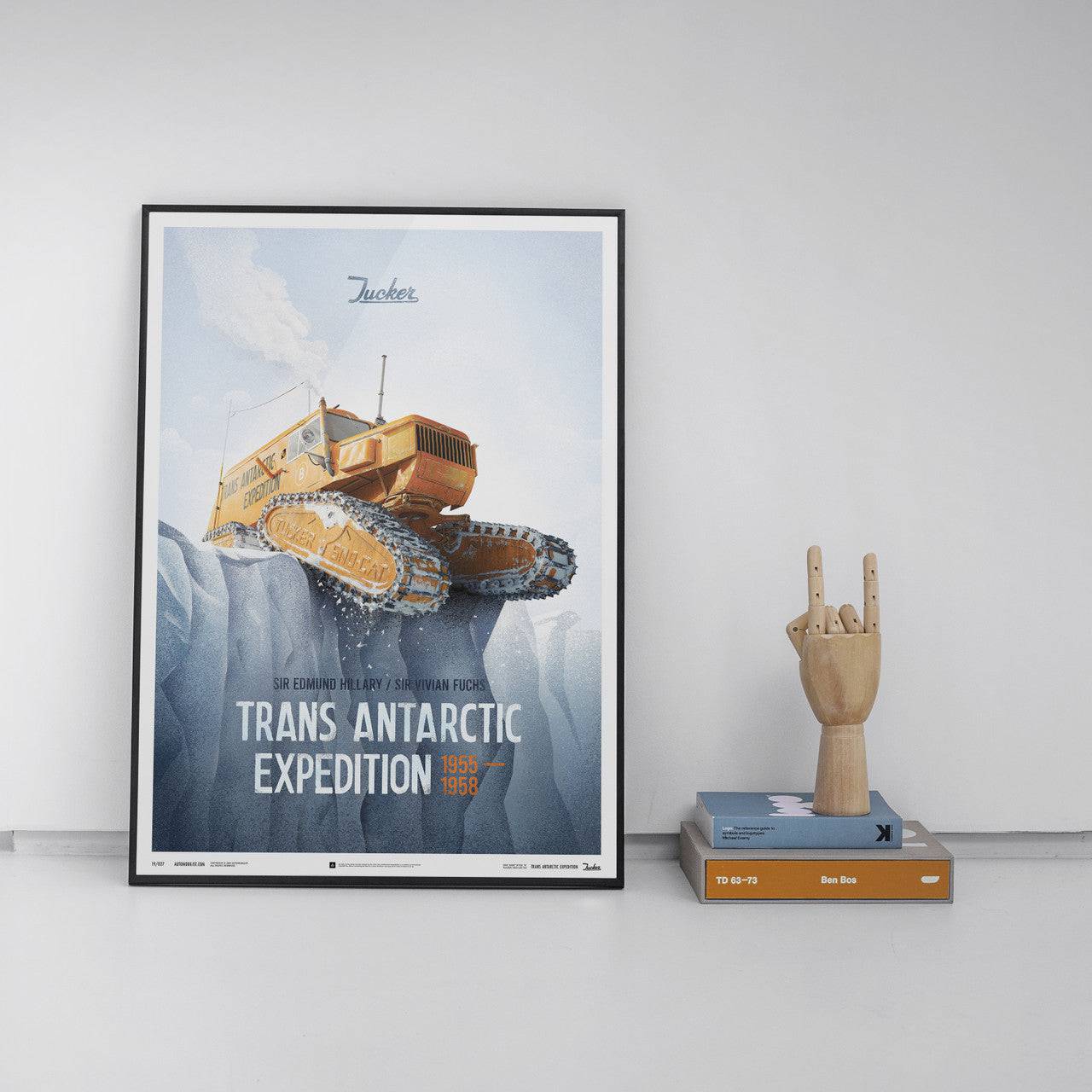The indoor photograph showcases a neatly arranged scene against a soft gray wall with a slightly darker gray baseboard and floor. Leaning against the wall is a narrow black-framed print with glass cover, titled "Sir Edmund Hillary and Sir Vivian Fuchs' Trans-Antarctic Expedition 1955-1958." The image within the frame highlights a massive orange expedition vehicle equipped with snow tracks, resting on a frozen iceberg. To the right of this framed print, two books with brown and blue spines are stacked on top of each other. Atop the blue-spined book is a wooden artist's hand model, with fingers positioned in a rock and roll devil sign.